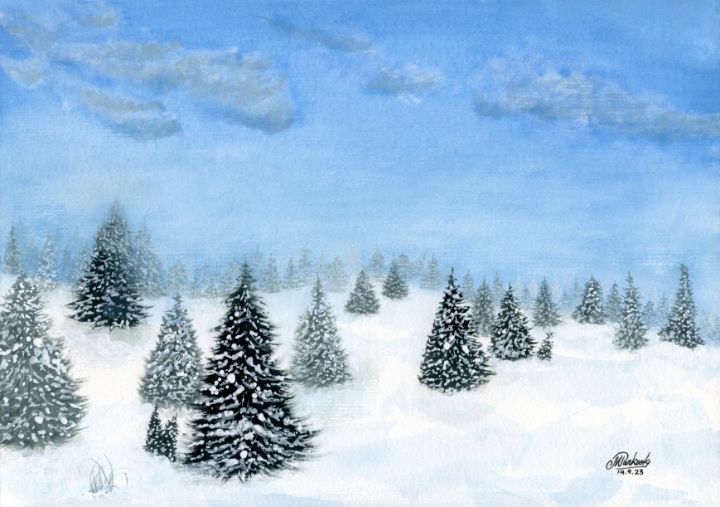The image, likely a greeting card illustration, features a serene winter landscape. The horizontal rectangular frame showcases an artist's signature in black cursive in the lower right-hand corner, accompanied by a date, "14-9-23." The foreground, occupying the bottom 40% of the image, displays rolling ground blanketed in deep snow, punctuated by a variety of conical-shaped evergreen trees. The trees, resembling Christmas trees, vary in size and saturation; some are darker green with sparse snow coverage, while others are lighter green, heavily laden with snow. In the distance, a faint line of evergreen trees marks the horizon, emphasizing their remoteness. The snowy terrain is depicted with varying shades of bright white and light blue, adding depth to the scene. Above the snowy landscape, the sky transitions from dark blue to lighter blue streaks, interspersed with a few scattered clouds, contributing to the overall hazy ambiance.